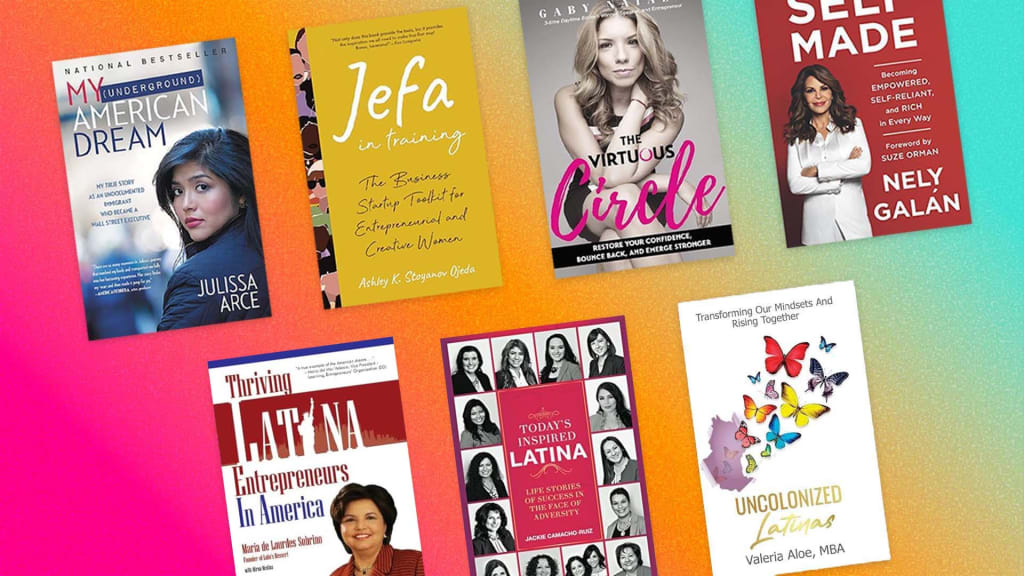The image depicts a stylized collection of seven book covers arranged on a slightly diagonal, upward angle from the lower left to the upper right. The covers are set against a grainy, colorful background that transitions from purple in the lower left to pink, orange in the center, and light blue in the upper right. In the top row, from left to right, the books are:

1. "My Underground American Dream"
2. "JEFA in Training: The Business Startups Toolkit for Entrepreneurial Woman"
3. "The Virtuous Circle" featuring a photo of a young woman
4. "Self-Made: Becoming Empowered, Self-Reliant, and Rich"

In the bottom row, from left to right, the books are:

5. "Today's Inspired Latina"
6. "Uncolonized Latinas"

The books vary in design, featuring both photography and text, and appear to focus on themes related to women's empowerment and Latina experiences. The cohesive arrangement and vibrant gradient background create an eye-catching and dynamic visual representation of the book covers.